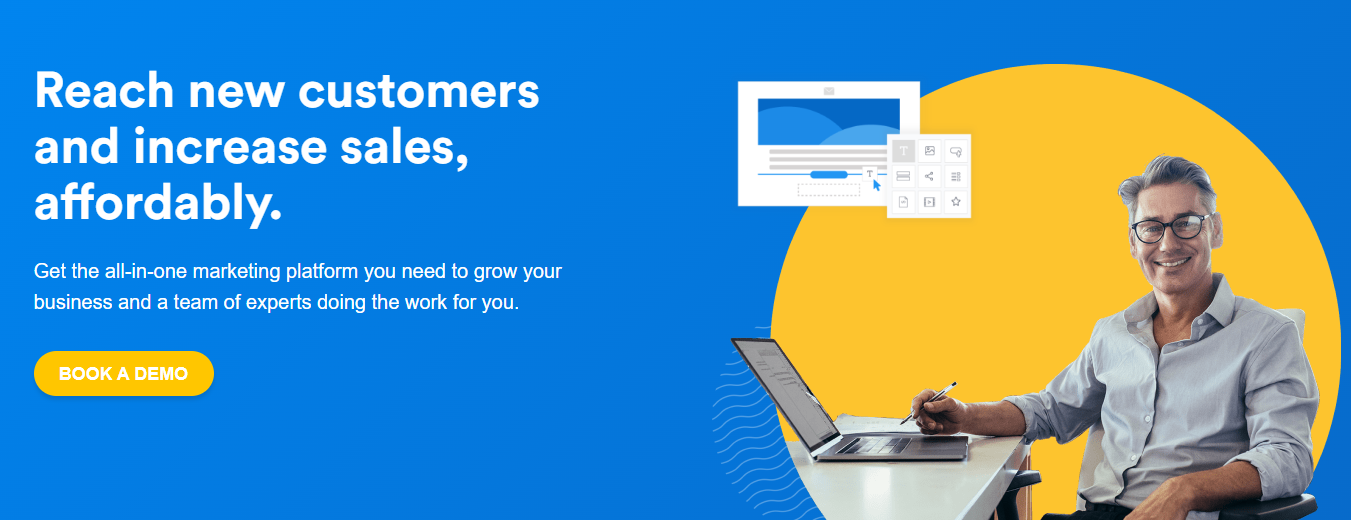This digital advertisement features a promotional message set against a blue background. On the left-hand side, white text highlights key benefits, stating: "Reaches new customers and increases sales affordably. Get the all-in-one marketing platform you need to grow your business and a team of experts doing the work for you. Book a demo." The right side displays an image of a middle-aged man seated at a desk with a laptop in front of him. He is turned slightly towards the camera, smiling, and holds a pen in his right hand. A large yellow circle serves as a vibrant backdrop behind him, emphasizing his presence. The overall design suggests the advertisement is for a comprehensive sales and marketing platform aimed at helping businesses expand their customer base and boost sales efficiently.